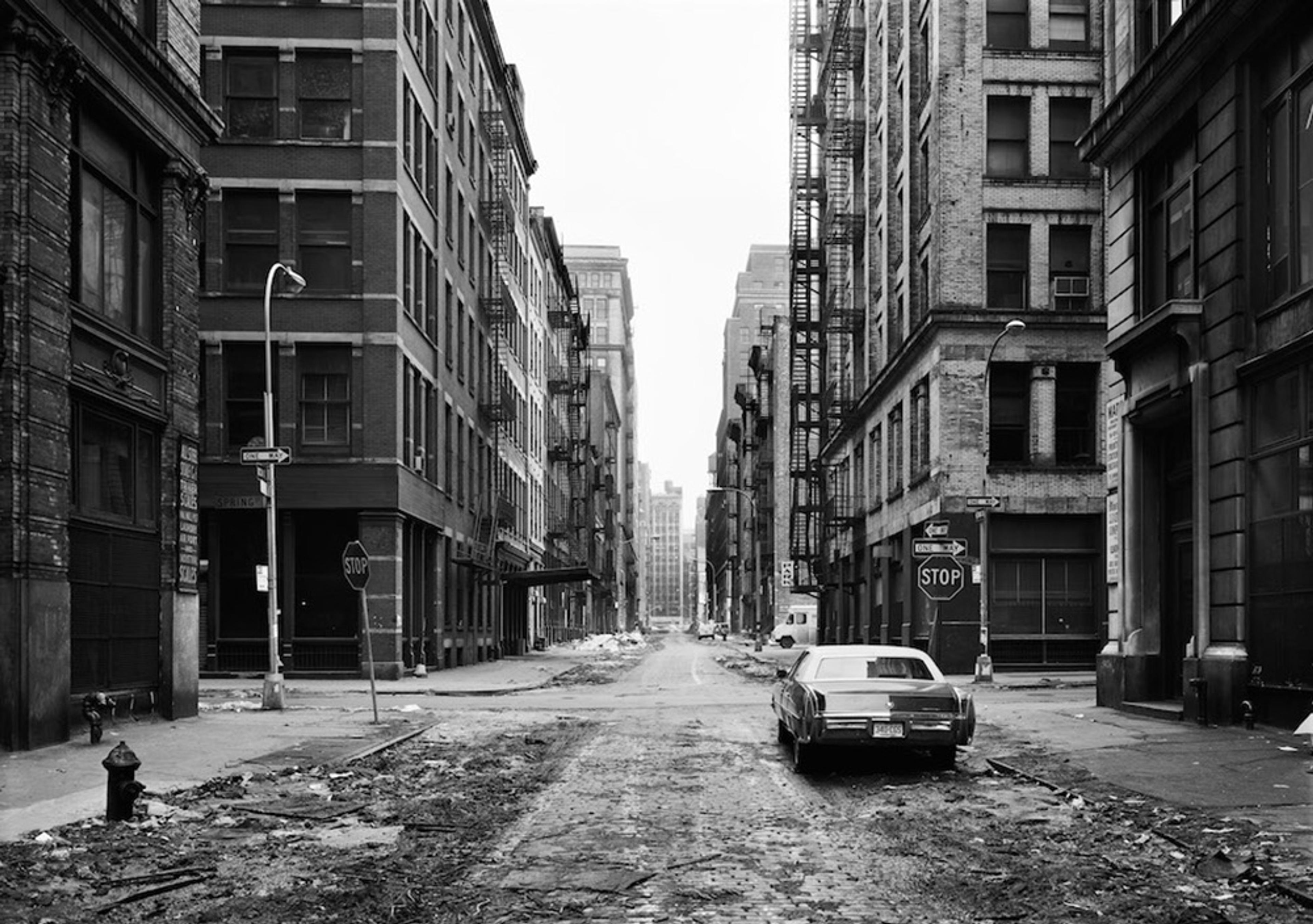This detailed black-and-white photograph captures a seemingly deserted city street viewed from its midpoint, flanked by tall, primarily brick buildings with emergency staircases. The street, which is in poor condition with visible debris, mud, and dirt, suggests recent neglect or turmoil. There are various street signs, including two stop signs on either side; the one on the left is bent, facing towards a building. One-way street signs point in different directions. A car is positioned in the foreground on the right side, its back end facing the camera, and a white bus can be seen farther up the street between two buildings. Additionally, a fire hydrant is visible in the lower left corner of the image, surrounded by debris, hinting at the possibility of a recent fire. Streetlights and lampposts line the sidewalk, while the sky appears uniformly white, indicating a cloudy day. The cars, and the modern-looking signage, suggest that the photograph might date from the 1960s or 1970s.